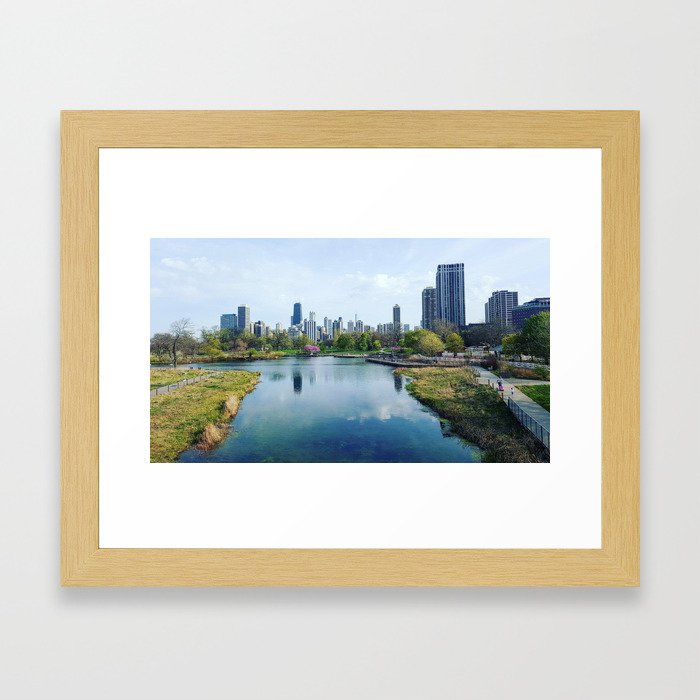This framed horizontal photograph, set with a natural wood finish and a wide white mat, captures a striking cityscape that appears to be of the Chicago skyline. The center of the image features a wide, bluish river, which reflects parts of the towering skyscrapers in the background, highlighting one particularly dominant building rising above the others. The scene is bathed in a light blue sky with white clouds, suggesting it is mid-spring. To the right of the river, a boardwalk, adorned with a fence, stretches through a park-like area with trees and greenery that overlap some of the buildings. Small figures of people can be seen walking along the boardwalk, adding life to the serene setting.